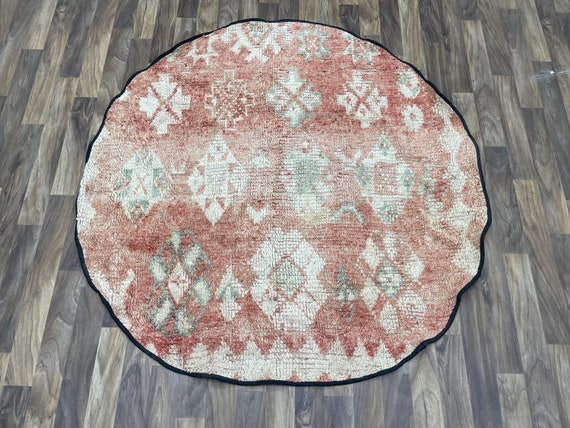The image depicts a circular rug positioned on a hardwood floor composed of dark and light wood panels, arranged in a distinctive parquet pattern. The rug features an Indian-style design with hues of wine red, faded to an almost salmon color, interspersed with greyish-green, white, and tan diamond shapes. Although the colors appear worn and muted, the intricate patterns remain discernible. A black trim accentuates the edges of the rug. The floor and rug both appear well-maintained despite the rug's aged appearance. There are no people or animals in the photograph, nor any identifying information to suggest its location.